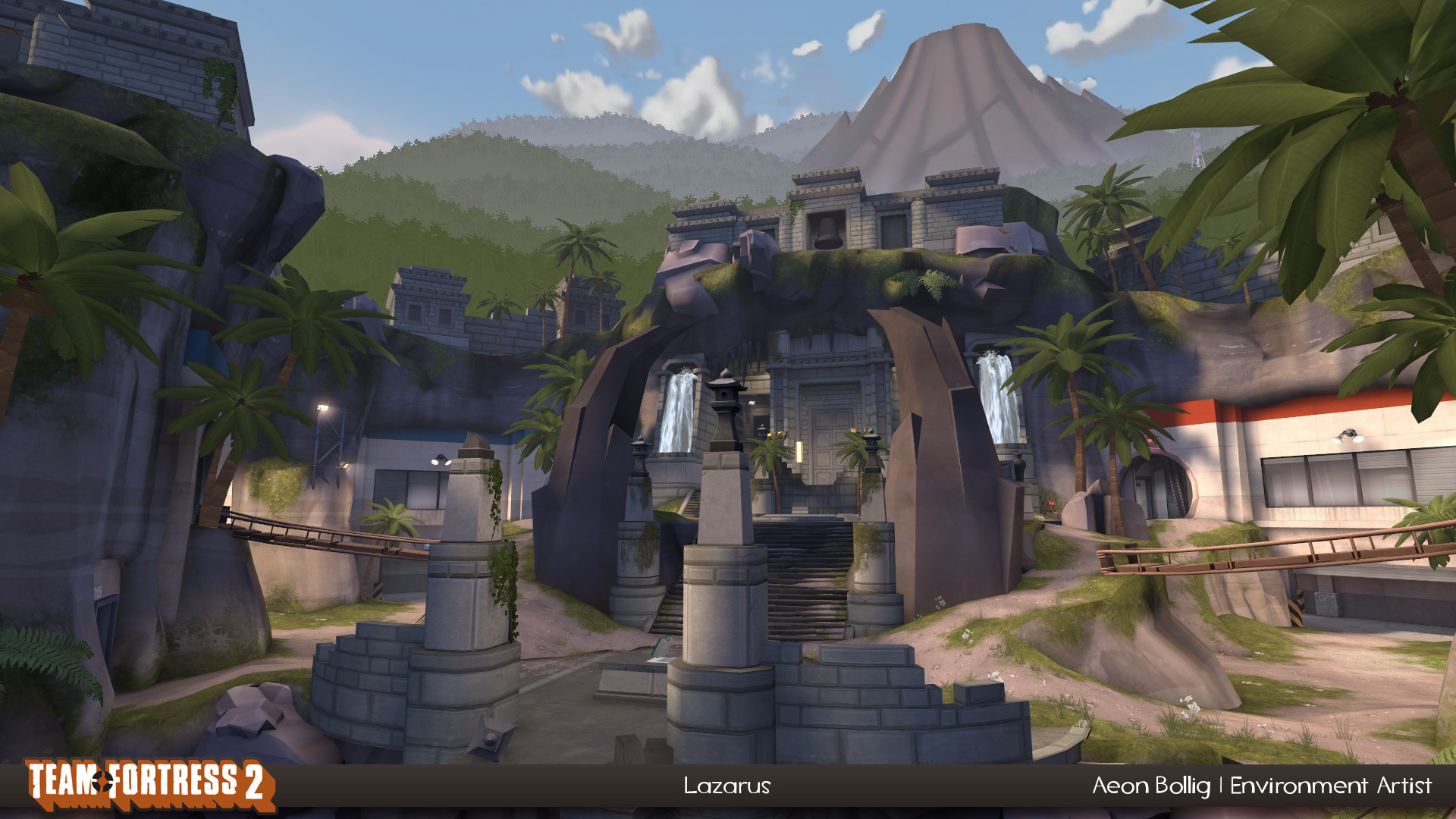This detailed, merged caption amalgamates the consistent and unique details observed by the different commentators. Here it is:

---

This image is a screenshot from the video game Team Fortress 2, with the game's logo evident in the bottom left corner in capitalized white letters with a reddish shadow. The level is called Lazarus, created by environment artist Eon Bollig, as indicated by text on the image. Central to the screenshot is the entrance to a large, uniquely-shaped grayish structure that appears to be a temple or castle. This building is accessed by a series of stone steps flanked by two sizeable palm trees and framed by twin white-blue waterfalls cascading down either side. 

To the left and right of the main entranceway, which features a prominent stone arch—a brown arch with green growth—there are modern, round doorways leading into a building with more contemporary windows. The foreground also shows ladders on both sides and wooden bridges that span small slopes. Additionally, the environment includes a bell tower located above a rocky outcrop that transitions to another level above.

In the background, there's an active volcano situated centrally along with lush, tree-covered hills stretching off to the left. The scene is bordered by tall, distant mountains and rolling green hills that lend a vibrant, natural backdrop to the central architectural focus.

---

This combined caption integrates the collective observations, emphasizing the recurrent themes and descriptive elements present in all three narratives.